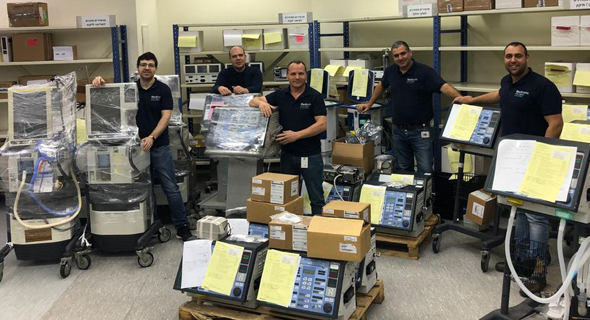The image depicts five men in a warehouse-like setting, all dressed in black polo shirts with a logo on the left side and jeans. They are surrounded by large electronic machines, some wrapped in protective plastic, possibly healthcare-related equipment. In the background, blue-framed shelving units filled with various items, including white-shelved sections, are visible, suggesting a well-stocked storage area. The men, who all have short hair, are leaning against different pieces of equipment and smiling at the camera, with one or two smiling more prominently. Boxes scattered around the room indicate readiness for delivery or inventory management, adding to the industrious atmosphere of the scene.